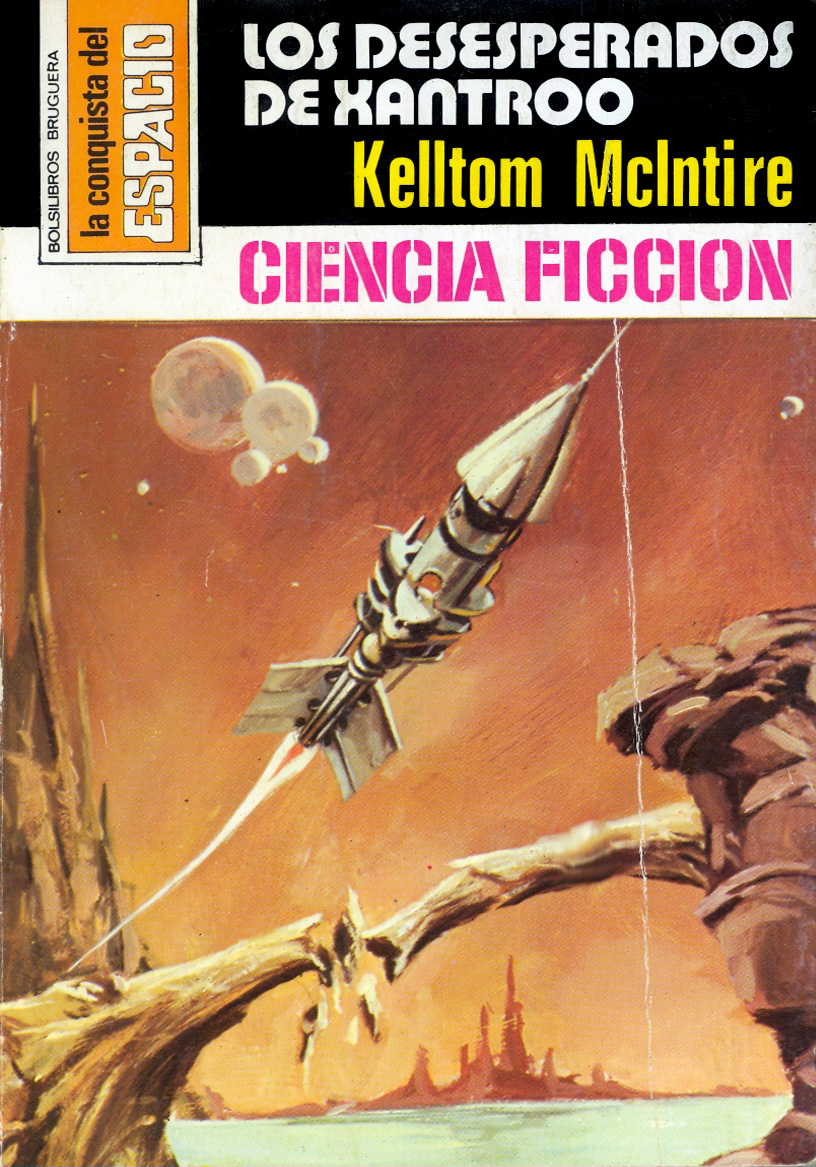The image is a captivating cover of a science fiction novel, written in Spanish, likely by US-based author Keltom McIntyre, titled "Los Desperados de Xantru." Dominating the forefront is an illustration of a white, black, and gray rocket, launching diagonally from the lower left to the upper right, piercing a surreal, alien sky painted in gradients of dark and light orange. The sky is adorned with multiple lunar bodies, suggesting an otherworldly setting. Below, jagged cliffs envelop the scene, with a broken tree branch dramatically positioned in the middle, possibly impacted by the rocket's liftoff. In the far background, a mountain range adds depth to the otherworldly landscape. The upper section of the cover features text on a black background, with vibrant white, yellow, and pink hues spelling out "Bocelabros Ruguerra, La conquista del Espacio," and "Ciencia Ficción," highlighting the novel's adventurous and extraterrestrial themes.